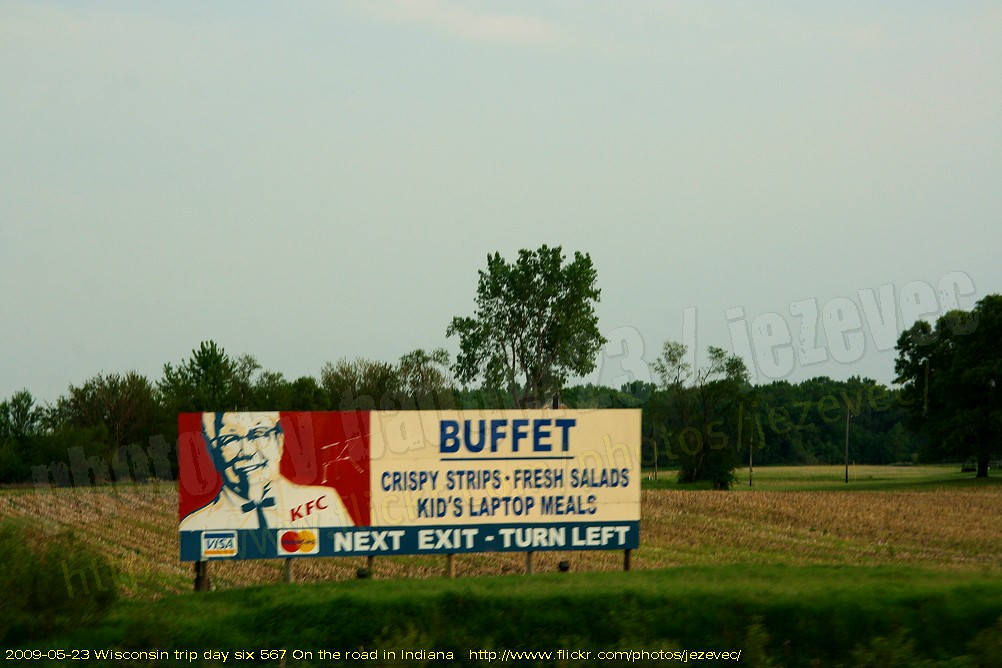In this photograph, we see a Kentucky Fried Chicken billboard prominently displayed in a rural setting. The billboard, which stands tall on six sturdy legs, has a red section on the left featuring the iconic image of Colonel Sanders. The right side has a white background with blue text advertising "Buffet, Crispy Strips, Fresh Salads, Kids Laptop Meals." Below this section, a blue strip advises travelers to take the next exit and turn left. In the foreground, a lush green hedge partially obscures the sign's base. To the left of the hedge, more greenery spreads out, creating a sense of depth and continuity. Beyond the billboard, a vast field stretches out with brown soil, eventually giving way to a line of green trees. The sky overhead is a clear, light blue, adding to the serene, open-road atmosphere of the image. At the bottom of the image, white text reads “2009-05-23 Wisconsin trip day 6567 on the road in Indiana,” followed by a URL: "http://www.flickr.com/photos/E-Z-E-V-E-C/."